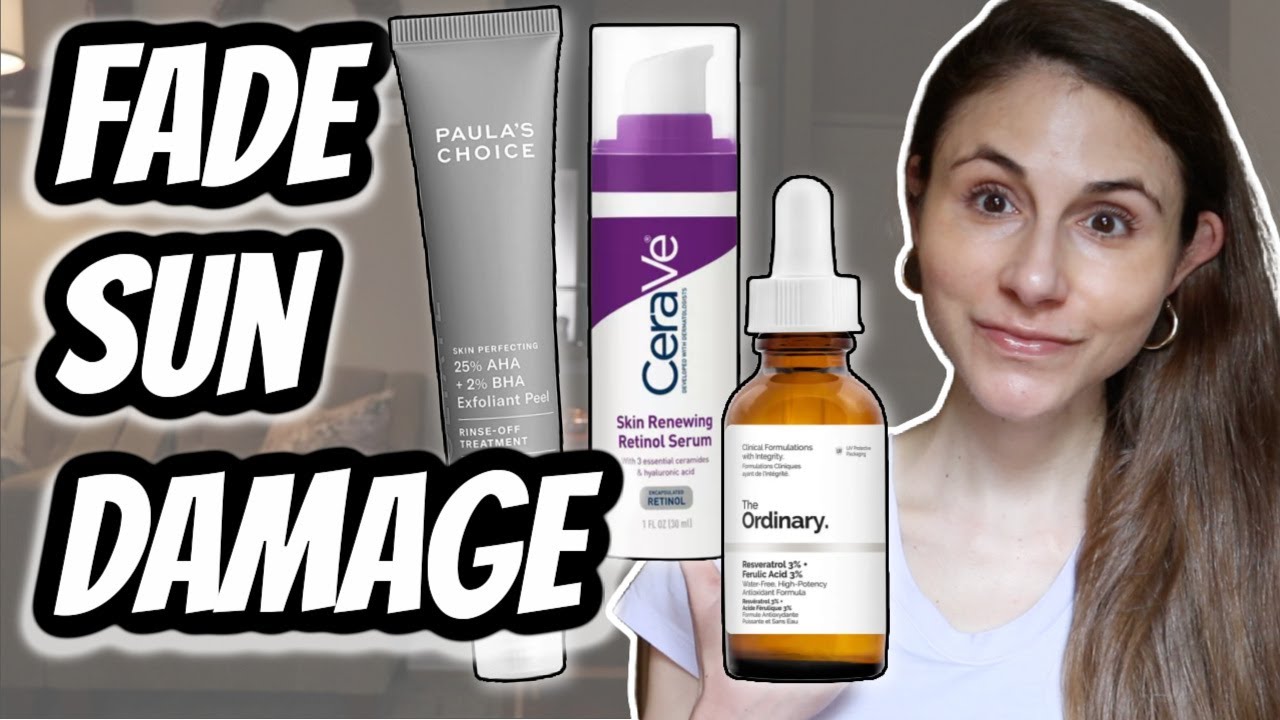The image prominently features the bold white text "Fade Sun Damage" arranged vertically with each word on a separate line against a black background. To the left of the text, there are three skincare products displayed. The first product is a light gray tube labeled "Paula's Choice" at the top, identified as an exfoliant peel. The second product is a tall, slender bottle of "CeraVe Skin Renewing Retinol Serum" with a dark purple cap and white lower half. The third item is a brown glass bottle with a dropper labeled "The Ordinary," known for its clinical formulations. On the right side of the image stands a happy-looking white woman with long brown hair extending beyond the picture’s bottom edge. She is wearing a white V-neck t-shirt and a gold hoop earring in one ear. Her eyes are wide open, she has raised eyebrows, and she is slightly smirking as she gazes at the products. The backdrop of the image is a grayish-brown faded depiction of a room.